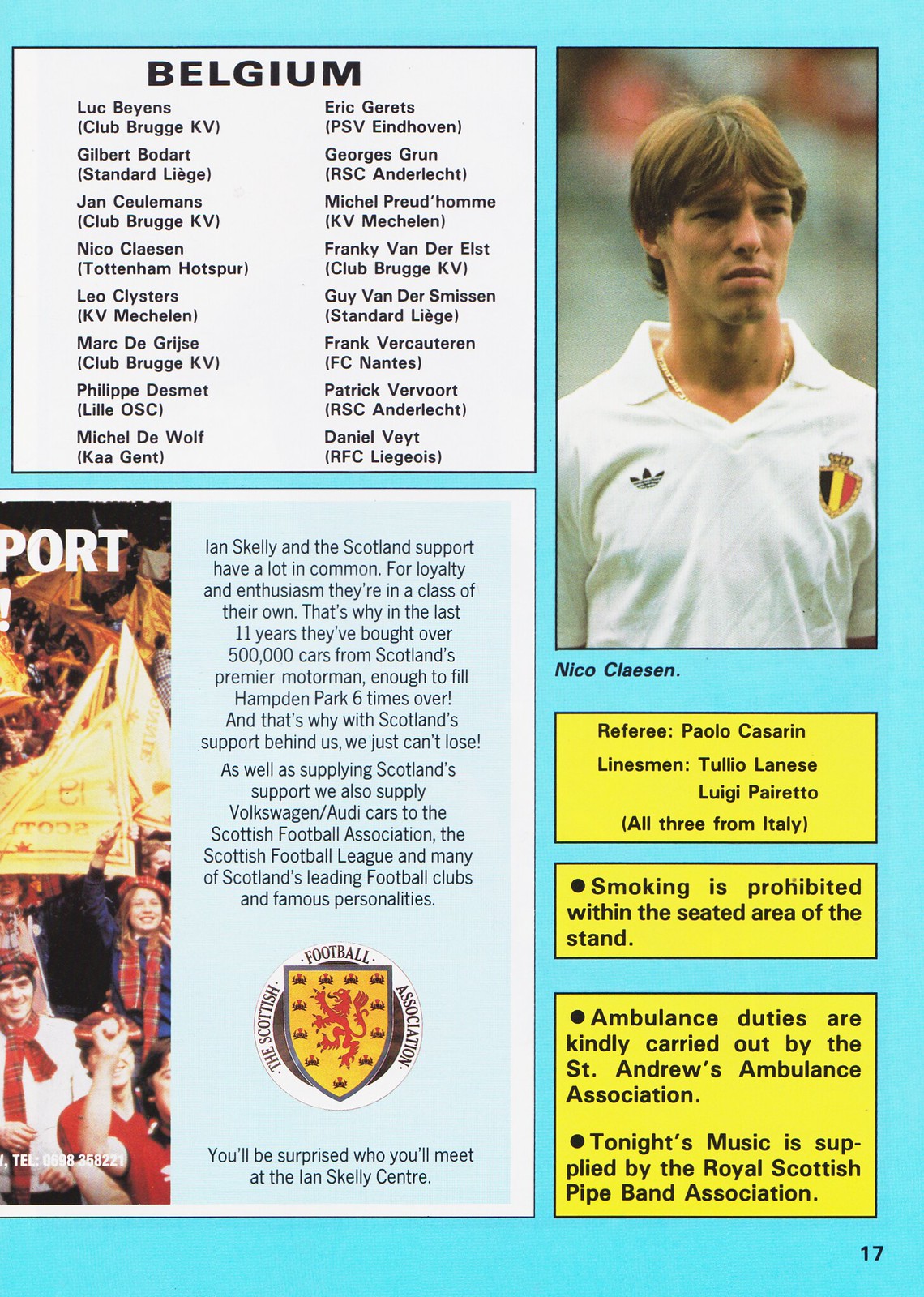This detailed caption combines the information from the various descriptions to provide a comprehensive view of the image:

"This image depicts a vintage football program page, featuring a blue background. In the upper left corner, a white square labeled 'Belgium' lists the names of players, including Luke Bevarose, Gilbert Bodart, and Juan Carlemans. Adjacent to this list is a color photograph of Nico Klaesen, a white male with brown hair, wearing a white polo shirt adorned with an Adidas logo on the right chest and a shield emblem on the left chest. Underneath his photo, it states 'Referee: Paolo Casarin; Linesmen: Tullio Laresi, Luigi Pernetto' – all officials from Italy.

To the right, a partially visible photo of a cheering crowd accompanies black text that extols Ian Skelly Centre's connection with Scottish football and its supporters. Below this text, a round logo of the Scottish Football Association is displayed, featuring a yellow shield with a red lion.

Three yellow squares sit below the advertisement, containing important notices in black text. The first square advises that 'Smoking is prohibited within the seating area of the stand,' while the lower squares detail that 'Ambulance duties are kindly carried out by the St. Andrews Ambulance Association,' and 'Tonight's music is supplied by the Royal Scottish Pipe Band Association.'

This array of text and imagery portrays an event between Belgium and Scotland, reflecting the themes of loyalty, enthusiasm, and historical context within the football community."